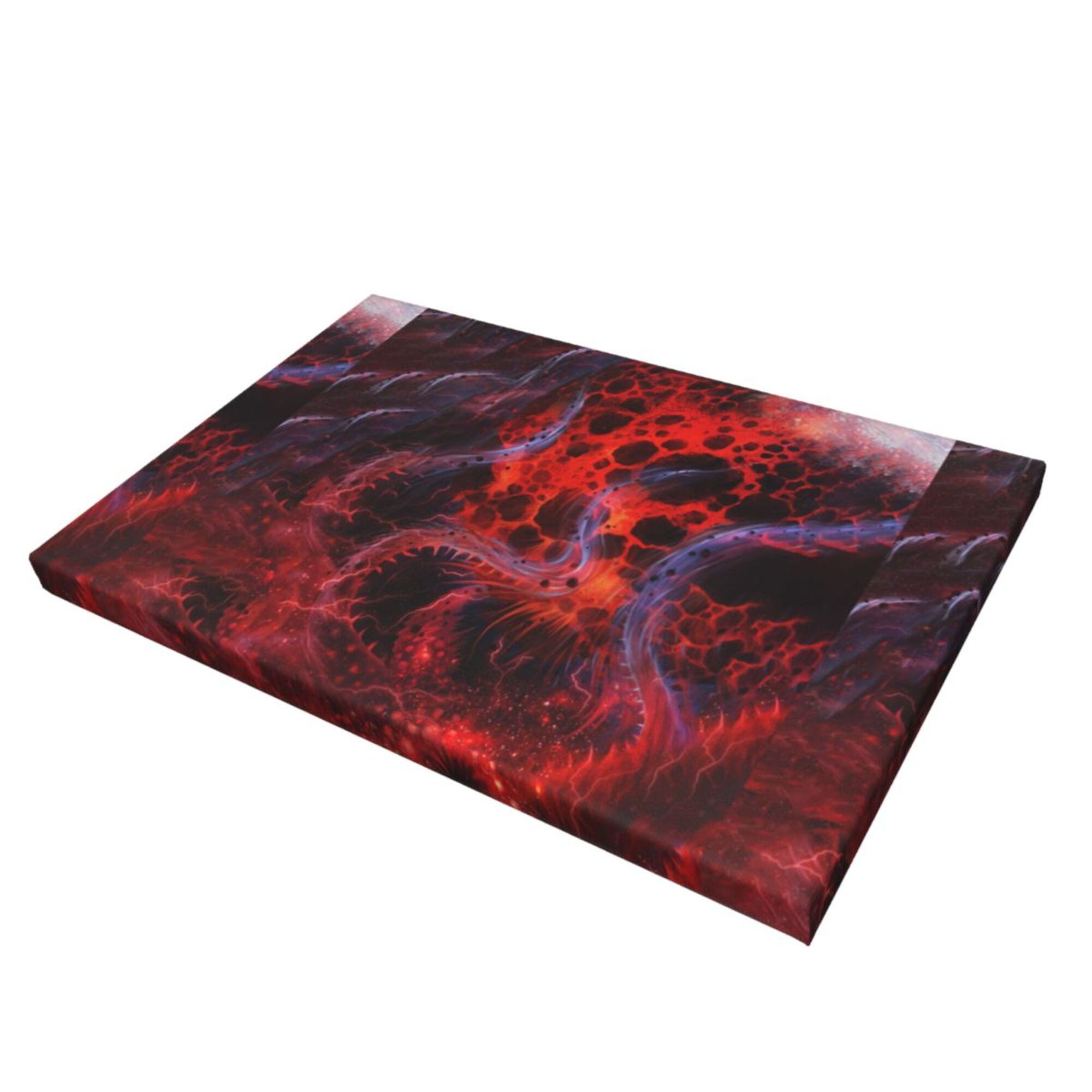This image depicts a box-like structure that resembles a painting on parchment, positioned at a slight angle to the right on a flat surface. The scene within the painting is surreal and otherworldly, featuring a vibrant, fiery landscape dominated by a molten red and orange lava background interspersed with smoky brown tints. Rising from the bottom of this chaotic environment are spectral gray, snake-like tentacles, adorned with spikes along their edges, evoking a sense of cosmic horror. The tentacles and the smoky vapor appear to be climbing upward amidst the tumultuous lava, suggesting an upward flow of energy and motion. The entire composition is bathed in glistening, violent hues of red, black, orange, and purple, creating an overwhelming sense of turbulent, volcanic activity. This intense and unique portrayal gives the impression of a fantasy or outer-space scene, captivating with its dynamic elements and vivid color palette.